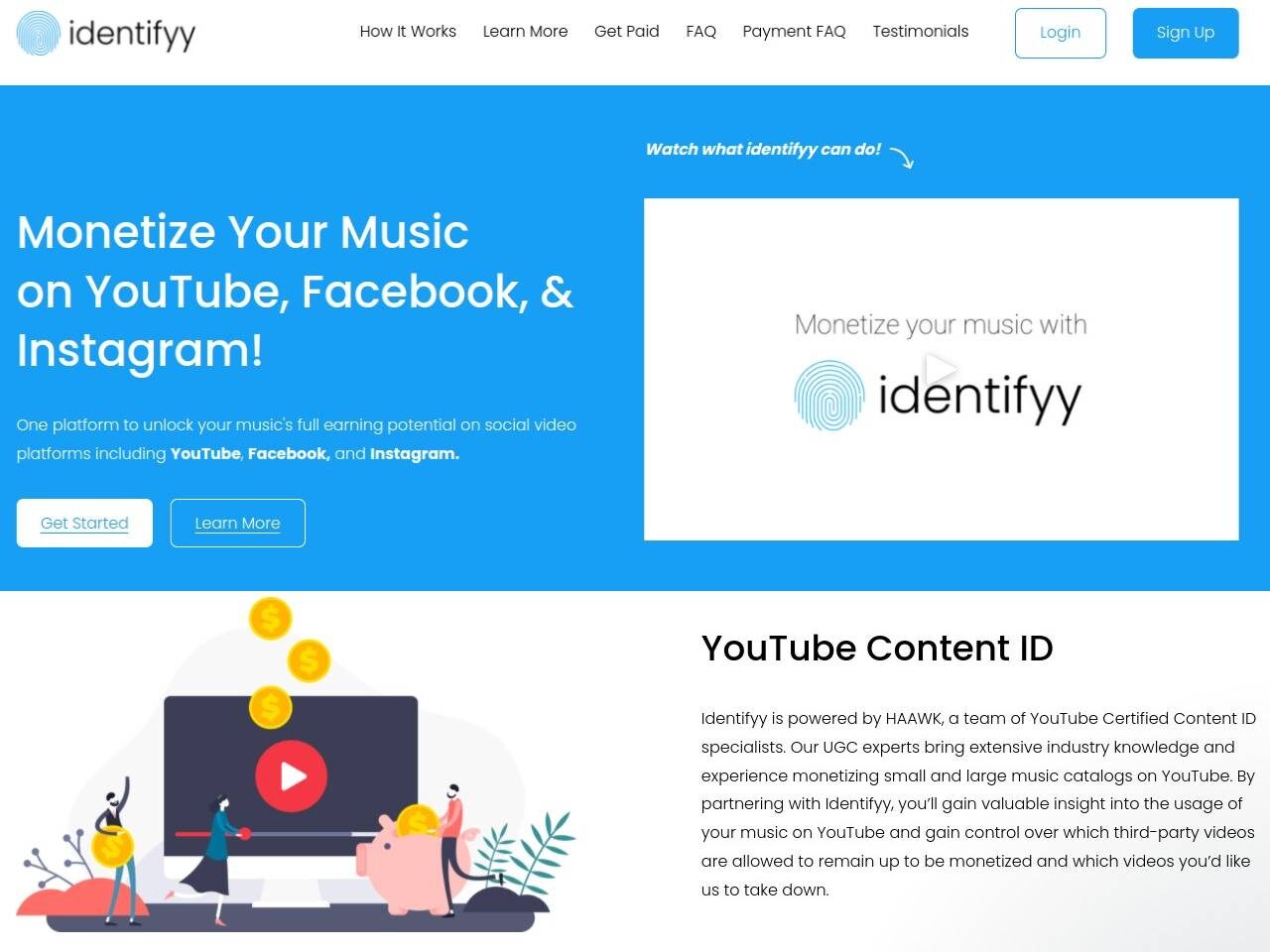The image showcases a music monetization website featuring a central thumbprint logo in the upper left corner, labeled "Identify" with a distinctive double 'I'. The main navigation menu includes options such as "How it Works," "Learn More," "Get Paid," "FAQ," "Payment FAQ," "Testimonials," a white "Login" button with blue text and border, and a blue "Sign Up" button with white text.

Dominating the page is a wide, tall blue banner with large white text on the left, proclaiming "Monetize your music on YouTube, Facebook, and Instagram!" Below this headline, additional text elaborates: "One platform to unlock your music's full earning potential on social video platforms including YouTube, Facebook, and Instagram." Beneath this description, two buttons are present – a white "Get Started" button and a blue "Learn More" button.

On the right side of the banner, a section invites users to "Watch what Identify can do," featuring a downward-pointing arrow towards a thumbnail box. This box includes a play button icon represented by a right-facing triangle, set against a ghosted backdrop. 

Farther below, a graphic illustrates the concept of monetizing music with Identify. The logo reappears alongside images of coins falling into what resembles a YouTube screen, where people are dancing and interacting with a desktop interface. A prominently large man is depicted placing a coin into an oversized piggy bank. To the right, text reads "YouTube Content ID," accompanied by a brief explanatory note in smaller print.